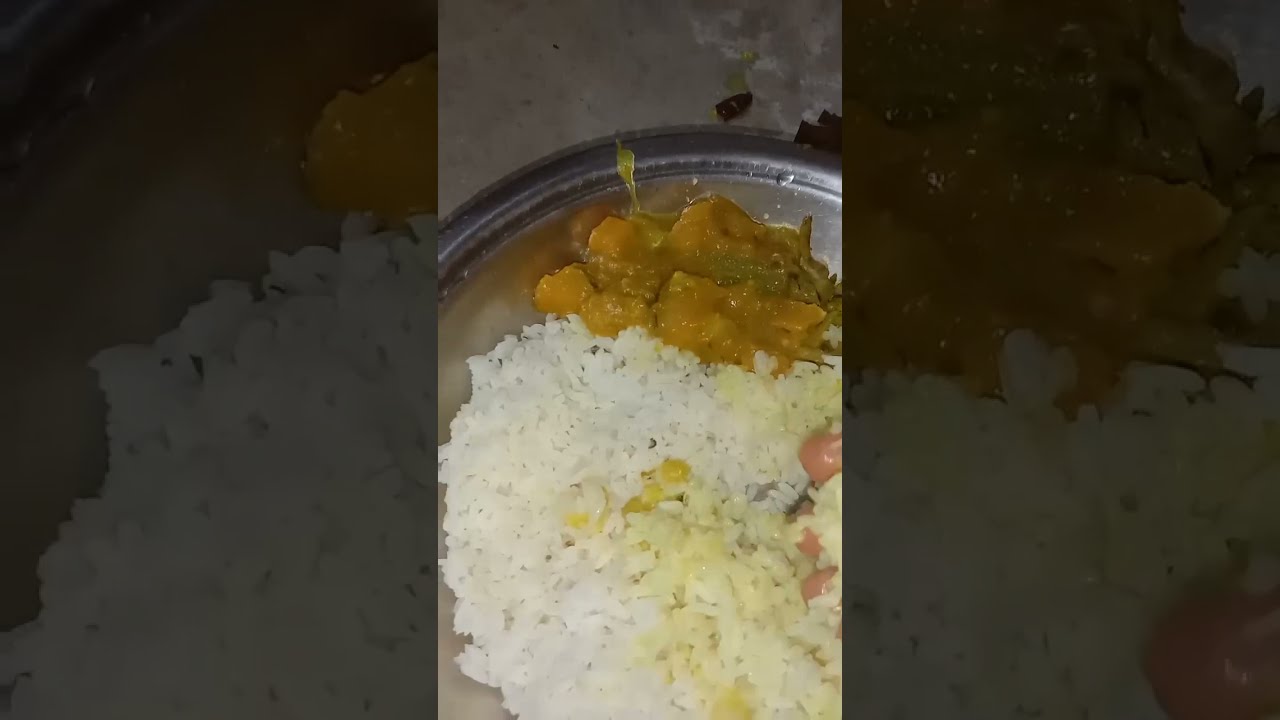The image is a vertical, smartphone-captured photograph, depicting a silver metallic plate resting on a dark gray surface, possibly marble or cement. The plate is prominently filled with a substantial amount of white rice, interspersed with dribbles of yellow and orange sauces. A portion of the rice is slightly discolored, suggesting the presence of melted butter. Accompanying the rice is a yellow-colored curry laden with chunks of vegetables, including potatoes and possibly some green and white elements typical of a vegetable dish. Additionally, there are a few pinkish onion-like objects on the plate. The lighting in the photo is poor, and the image isn't entirely clear, though the details of the food are discernible.